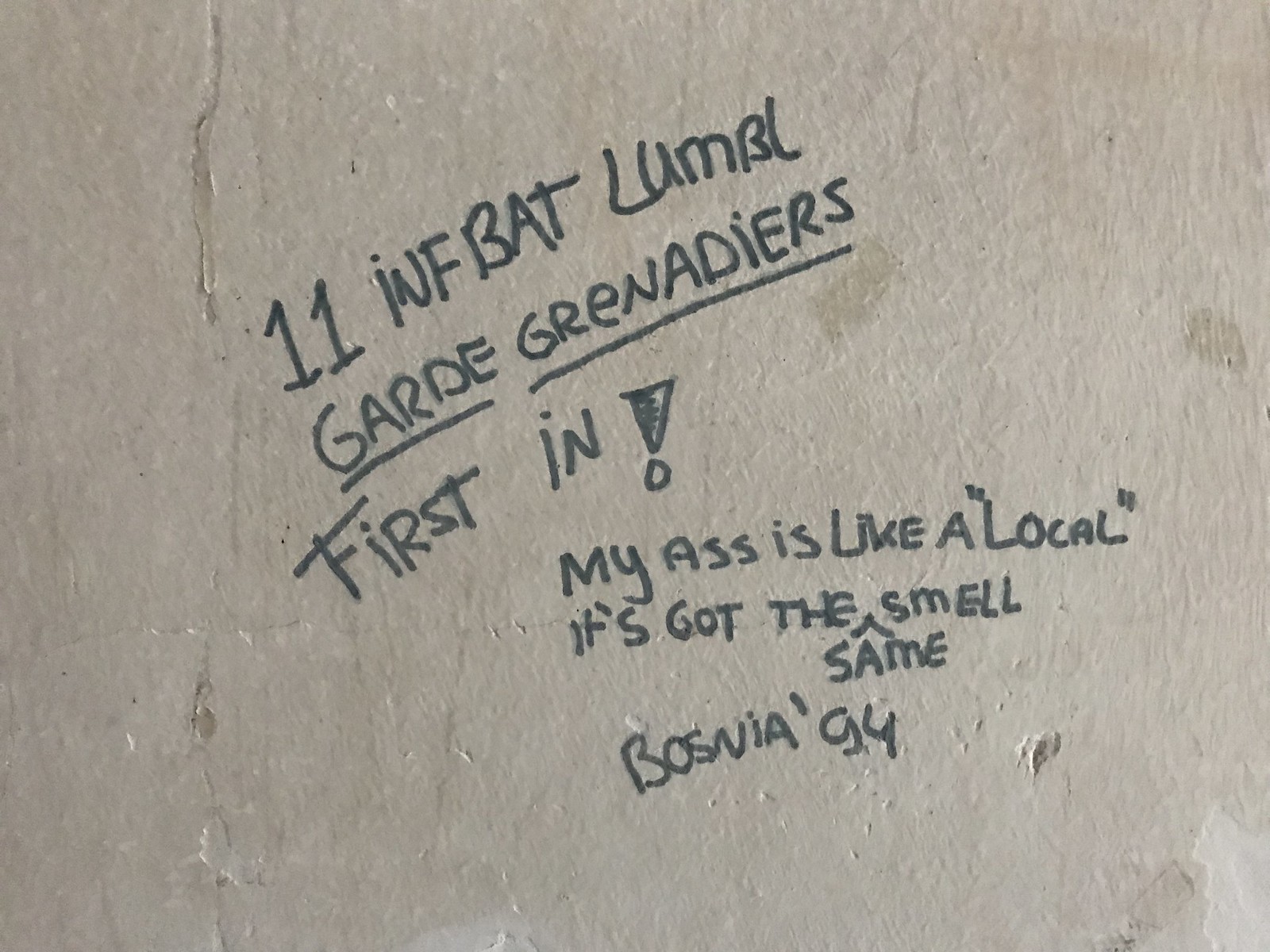The image depicts a light brown, graffiti-covered wall with a vertical crack running down the left side. The wall, made of stucco, shows signs of wear with pits, holes, and stains scattered across its surface. In the center, written in black marker, there are two distinct sections of text. The first section, slanted upwards towards the right corner, reads: "11 INFBAT MLUMBO GUARD GRENADIERS FIRST IN!" The '!' is formed with an upside-down triangle and a dot. Below it, another paragraph written horizontally states: "My ass is like a loco. It's got the same smell. Bosnia '94." This graffiti appears to reflect sentiments from a past military conflict, capturing a moment in time on this worn wall.